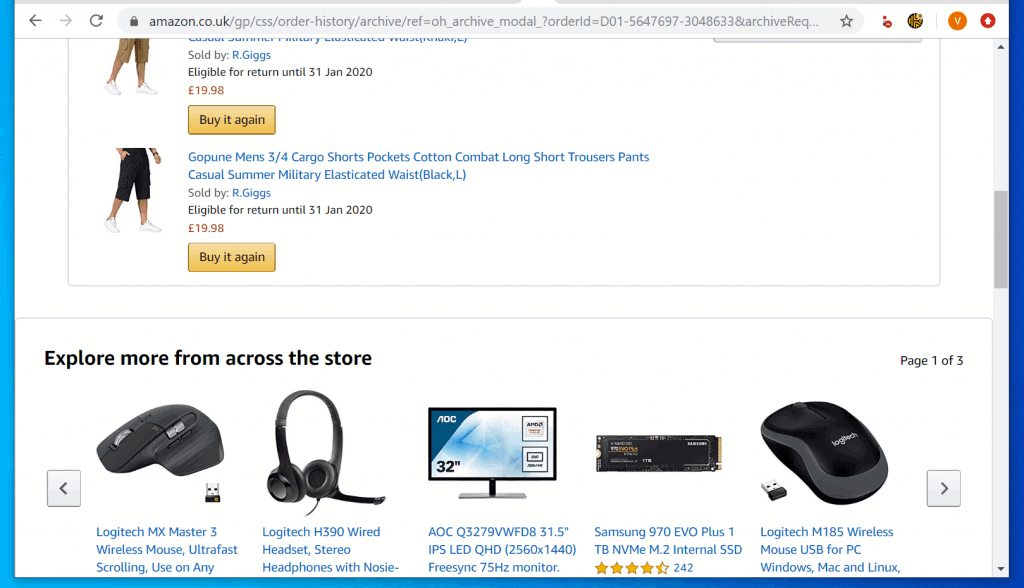A detailed screen capture of an Amazon webpage is displayed, showing several elements. At the very top, there is a gray address bar with navigational buttons—back arrow, forward arrow, and refresh icon—alongside a padlock icon. The URL begins with "amazon.co.uk" followed by a lengthy address. Further along, there are icons: a gray star, a red dot, an orange icon with a "V," and a red and white icon. 

The main content area of the webpage is set against a white background. The first item displayed is a pair of tan capri pants paired with white shoes. The listing states, "Sold by Our Gigs," and indicates that it is "eligible for return until 31st of Jan 2020," priced at 19.98 pounds. There’s a gold "Buy it again" button beneath this item. 

Following that, there is a listing for black capri pants, labeled as "GQ Poon Men's Three-Fourth Cover," described as "short pockets, cotton combat long short trousers, casual summer military elasticated waist, black large," also sold by "Our Gigs" and eligible for return until 31st of Jan 2020, priced at 19.98 pounds. This item also features a "Buy it again" button in gold.

At the bottom of this section, a black text header reads, "Explore more from across the store." Underneath, several products are showcased: a black Logitech mouse, a pair of black Logitech headphones, an AOC computer monitor, a Samsung Plus internal SSD with 242 ratings, and another black Logitech mouse.

Towards the bottom right corner of the display, there is a gray box with an arrow, indicating "Page 1 of 3." The entire image is framed by a blue border.